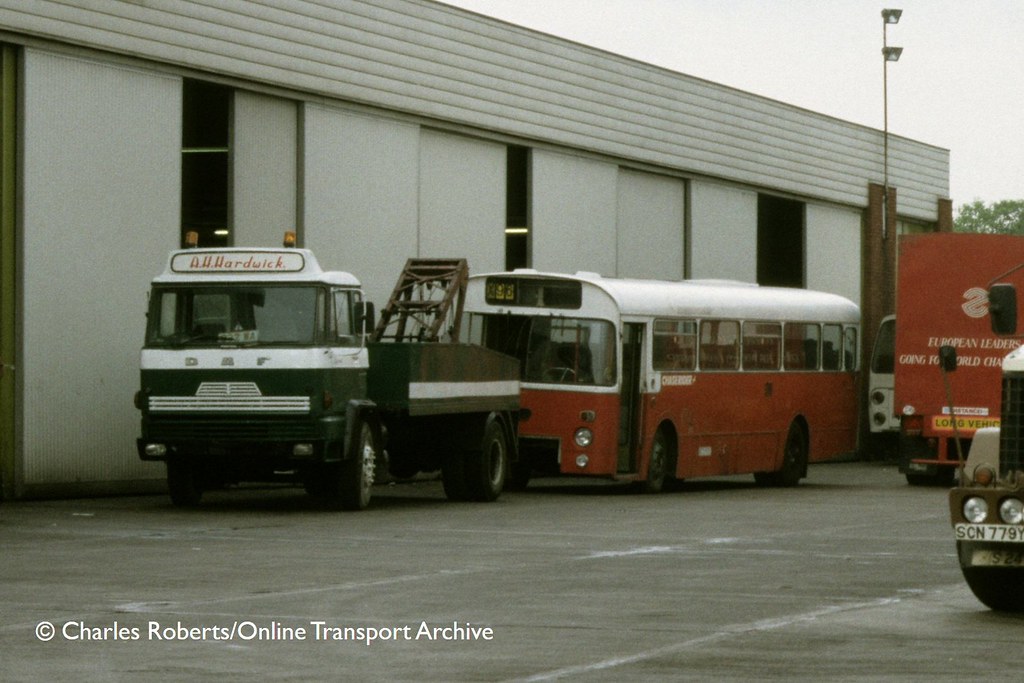The image depicts an outdoor scene beside a large, rectangular gray building, likely a factory or warehouse with shutter doors and some visible interior lighting. In the middle of the picture, parked along a gray concrete road and in a media parking area, is an old red and white bus marked with the number 96 at the top. Positioned in front of it is a green tow truck with white striping, a cable prepared to hook the bus, and an AH Hardwick sign in red font. Just behind this bus, another similarly sized vehicle can be partially seen. Toward the right side of the image, another red truck can be observed, bearing the phrase "European Leaders Going Forward and World Change" with a "Long Vehicle" sign at the bottom, all beneath a logo resembling an inverted S. Further to the right, a portion of another vehicle, a Mack truck with a white hood, greenish bottom, and the license plate SCN 779Y, is visible, along with its rearview mirrors and headlights. The scene includes trees and a clear sky in the background. The bottom left corner of the image features a watermark stating "Charles Roberts Online Transport Archive."